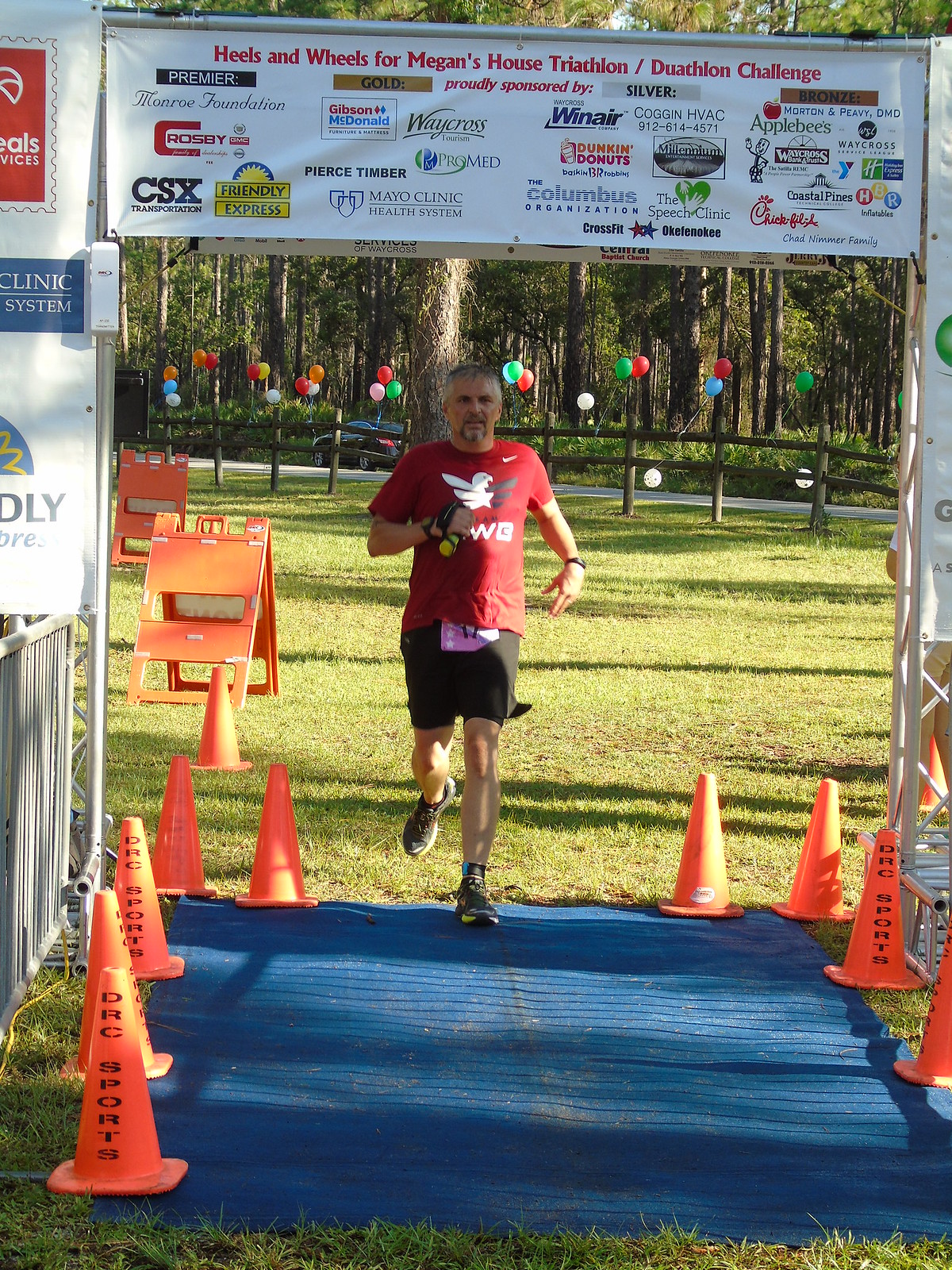The image captures a middle-aged man crossing the finish line of the "Heels and Wheels for Megan's House Triathlon/Duathlon Challenge." The scene is set on a grassy area with an organized event layout. The man, who appears to be in his 40s or 50s, is wearing a red t-shirt and black shorts, complemented by black running shoes. He has short, salt-and-pepper hair, a French beard, and is equipped with a running watch and fitness band. His race number is pinned to his shorts, and he holds a water bottle in his right hand. A blue finishing mat adorned with orange cones guides the participants to the finish, marked by a prominent banner overhead listing various sponsors. The banner prominently features names like Premier, CSX, and Aaron Day Express, along with numerous other logos and brand names. Multicolored balloons (red, blue, green, and white) tied to a wooden fence in the background add a festive touch, while additional orange banner stands and a parked car can be seen further behind. The event appears to be well-coordinated, with clear pathways and fencing to direct participants towards the finish line, amidst a scenic backdrop of green trees and pleasant weather.